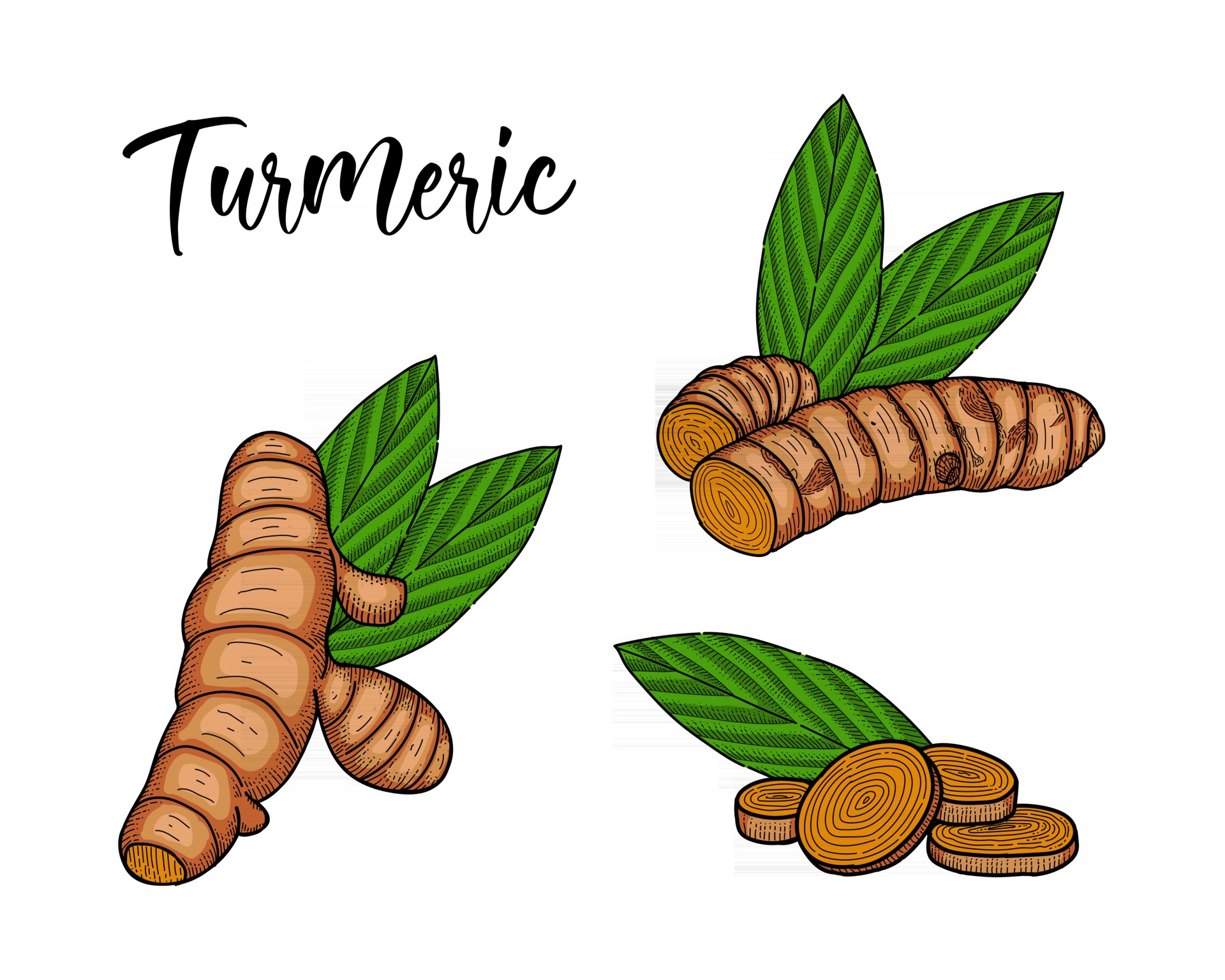This detailed color illustration of turmeric, set against a pristine white background, features the word "turmeric" elegantly inscribed in black script in the top right corner. Depicted are three distinct views of the turmeric root, all accompanied by its characteristic green leaves.

On the left, we see the whole turmeric root, prominently displayed with two green leaves showing a patterned blend of light and dark green that fan out in a V-shape. This whole root features several bulbous offshoots on its right side. 

To the top right of the image, a segment of the turmeric root is illustrated, partially cut to reveal its intricate, tree-ring-like interior. This segment, cut into a smaller piece at the tip, also displays the same two pointed green leaves.

Below this cut segment, in the lower right corner, four round slices of turmeric root are stacked, showcasing the vibrant, layered interior. These slices are accompanied by a single dark green leaf jutting out to the side.

This illustration captures the essence and details of the turmeric root and its leaves with a clean and vibrant style.